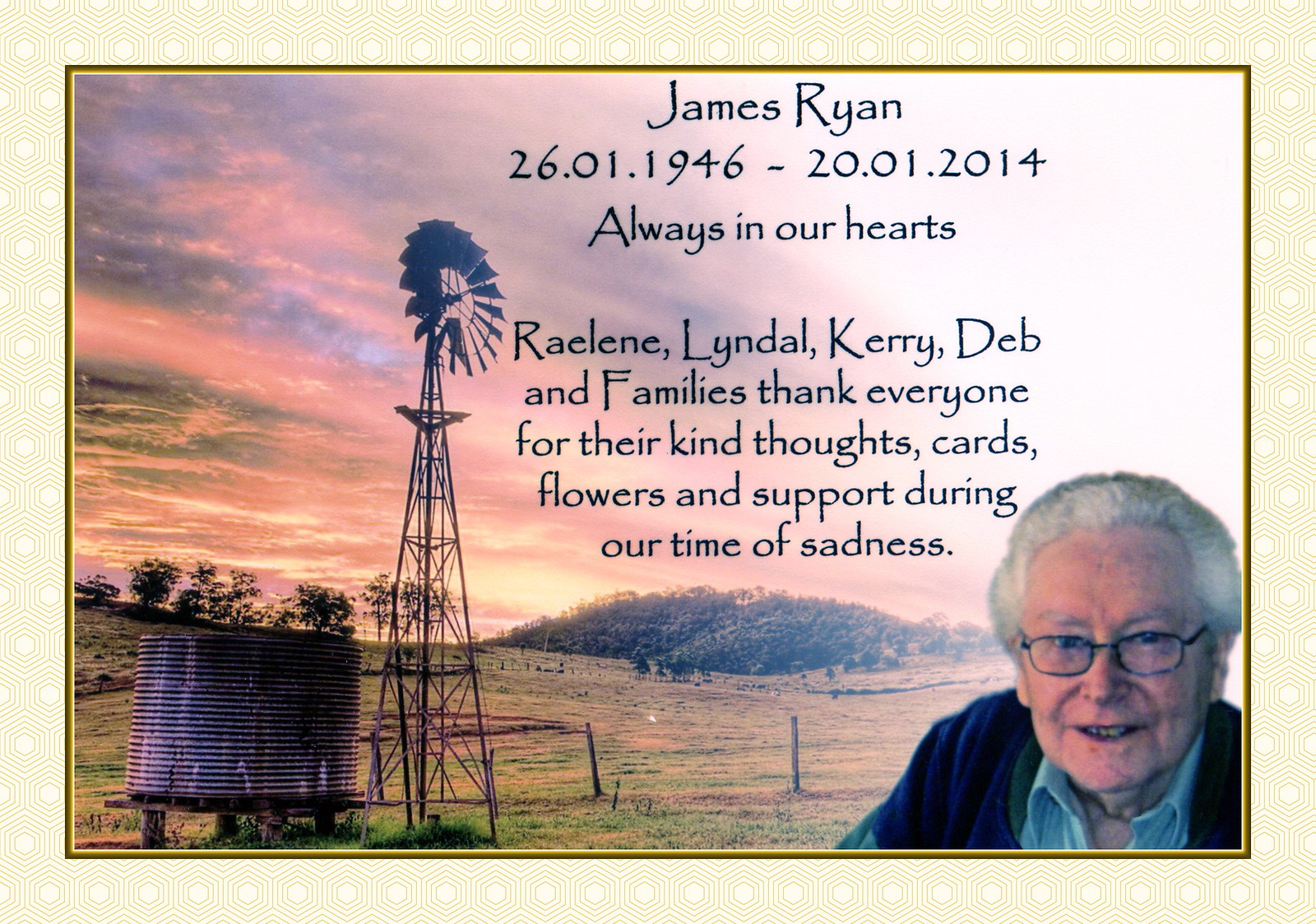The memorial collage image features a farm scene with multiple green hills, posts, and a barbed wire fence. A water well made of corrugated metal is situated next to a windmill in the foreground, under a twilight sky. The outer edges are framed with a hexagonal yellow line pattern. Centered at the top, text reads: "James Ryan, 26-01-1946 to 20-01-2014. Always in our hearts." Below, additional text in blue states: "Merlene, Lyndall, Carrie, Deb, and families thank everyone for their kind thoughts, cards, flowers, and support during our time of sadness." In the bottom right corner, there is a photograph of an elderly man with gray hair and glasses wearing a blue sweater over a collared shirt, presumed to be James Ryan. The detailed farm scene could be suggestive of James' own farm.